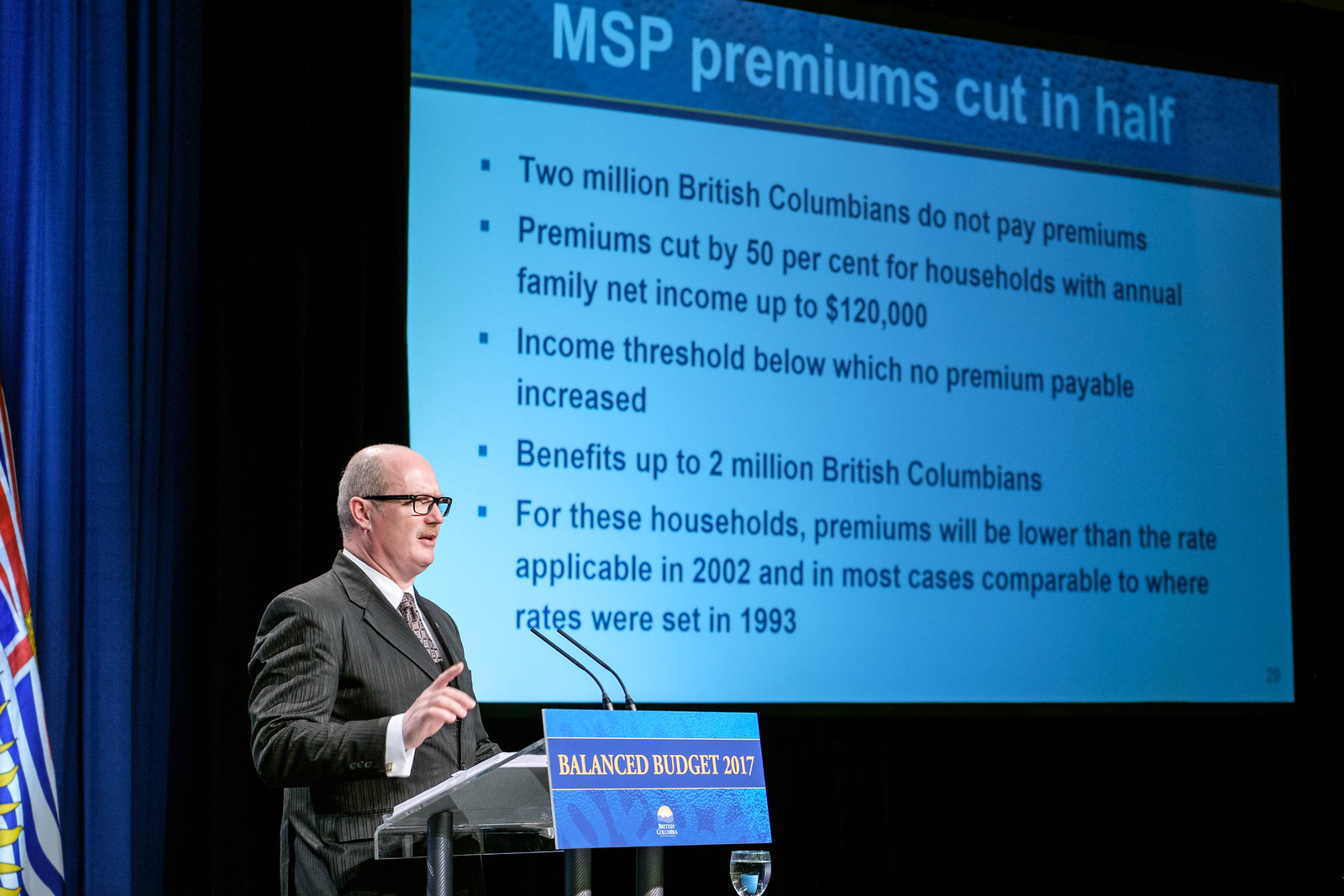This is a full-color, indoor photograph taken at a lecture, without any borders. The image features an older gentleman, possibly British, in a gray suit, bald and wearing black glasses, giving a lecture from a podium. His left hand is raised in the air. The podium has a placard that reads "Balanced Budget 2017." Behind him, a large screen displays details about MSP premiums being cut in half. The text on the screen also highlights that 2 million British Columbians do not pay premiums, with cuts of 50% for households with an annual net income up to $120,000. The screen further mentions an increase in the income threshold below which no premium is payable, benefits affecting up to 2 million British Columbians, and that for many households, premiums will be lower than the rates in 2002 and comparable to those in 1993. In the lower-left corner of the image, there is a flag resembling the Union Jack, suggesting a connection to a colony or former colony of England. The lecturer is discussing the implications of this new law on the MSP premiums.